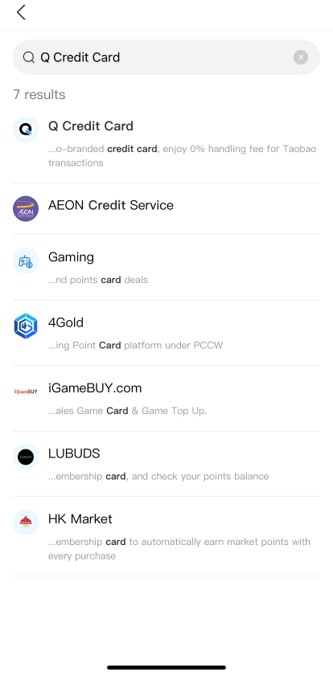This image depicts the search section of a website featuring an intelligent search function. At the top, there's a search bar with a subtle gray shading, accompanied by a magnifying glass icon. To the left of the search bar is a back button, designed as a simple line resembling a Pac-Man mouth. Below the search bar, the user appears to have searched for "Q credit card," which has yielded seven results. 

These results are listed in detail, starting with "Q credit card," which is marked with an icon. The description for this result reads: "Oh branded credit card, enjoy 0% handling fee for Taobao transactions." The subsequent results include "Aon credit service," "The Gaming Hub," "Goldfinch Finances," "igamebuy.com," "Lubuds," and "HK Market." Each result is accompanied by a uniquely colored icon, likely representing their respective brands or services. The search results suggest that the site caters to users interested in financial services, gaming, and online shopping, possibly targeting an audience in China or other parts of Asia.